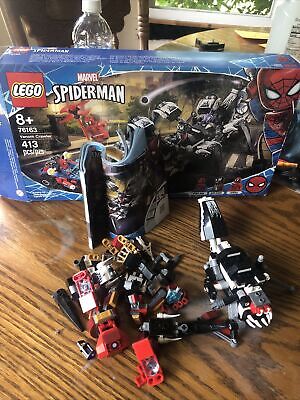This indoor photograph captures a busy scene on a medium brown wooden table, which features a partially assembled Lego vehicle surrounded by a scattered pile of multicolored Lego pieces, including gray, white, red, and yellow. To the right of the Lego pieces is a partially or fully assembled Lego vehicle. Directly behind the pile sits a booklet, which may be an instruction manual or another magazine. Dominating the center of the image is a large blue Lego box detailed with vibrant cartoon imagery. The box prominently displays the Marvel and Spider-Man logos along with the Lego branding in a red square. It also indicates the set is suitable for ages eight and up and consists of 413 pieces. The box’s illustration shows a Lego vehicle launching a boulder at a Lego Spider-Man, with an enlarged image of Lego Spider-Man on the right side. Behind the box, a plastic water bottle with a white cap peeks out, and a chair is partially visible to the left. A window in the background reveals a glimpse of green leaves, adding an element of natural light to the scene.